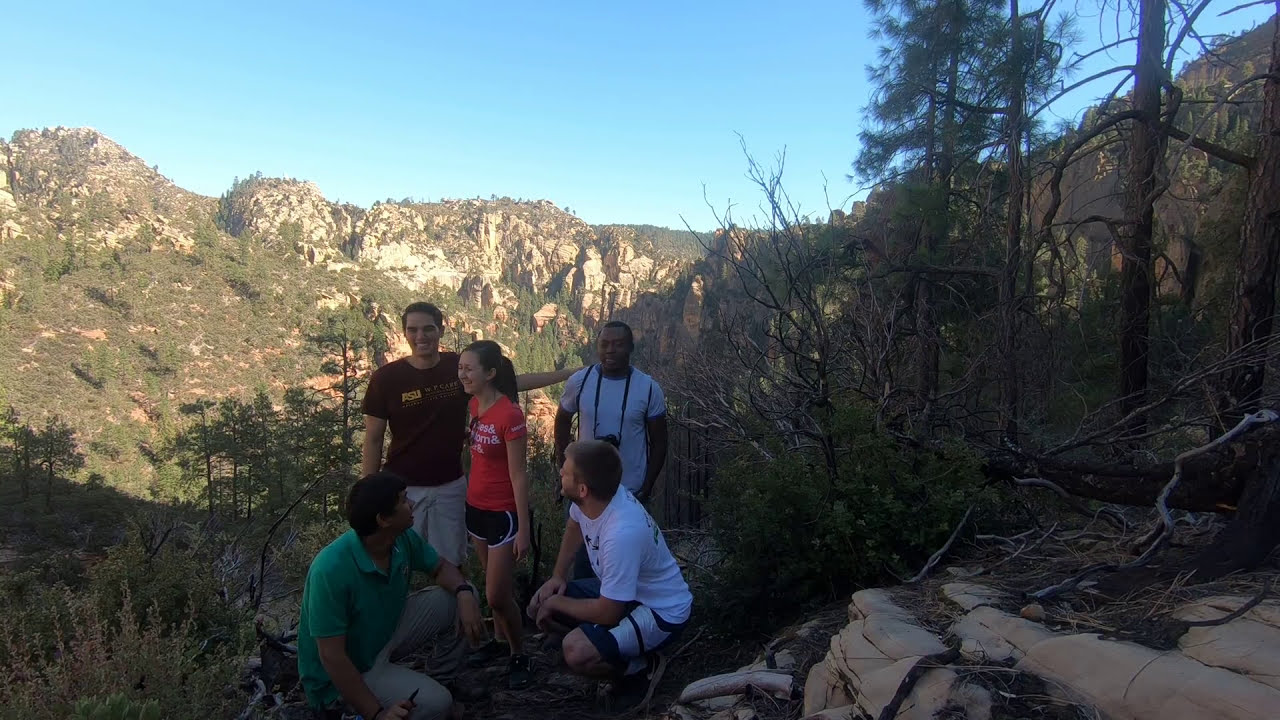This wide rectangular photograph captures a group of five young adults enjoying a hiking expedition on a rocky hill with a scenic backdrop of a sunlit mountain range covered in green trees and tan-gray rock formations. The clear, cloudless blue sky dominates the top of the image, providing a bright, natural light that enhances the vivid details of the landscape. In the bottom middle of the photograph, the group is positioned slightly to the left.

From left to right, we see the first man kneeling, an Indian male with black hair, wearing a green polo shirt and gray pants, looking back towards the group. Behind him stands another man, possibly Hispanic, dressed in a brown t-shirt and gray shorts. To his right stands a young girl with dark hair, in a red short-sleeve t-shirt and black shorts. To her right, a black male wearing a light t-shirt has a camera hanging around his neck. In front of him, kneeling down and facing left, is a white male with brown hair and a beard, dressed in a white t-shirt and blue and white shorts. The rocky surface they're gathered on is peppered with dirt and branches, leading into a densely wooded green area in the backdrop.

The image exudes a sense of outdoor adventure, camaraderie, and the joy of exploring the natural world.